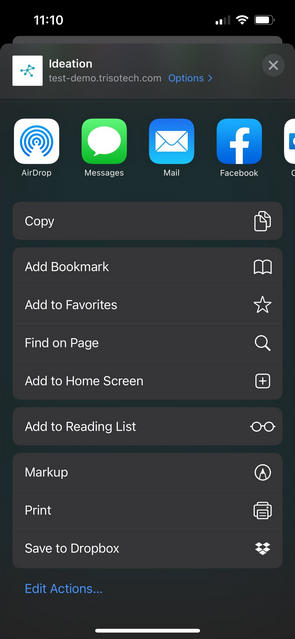The image is a screenshot from a mobile device, displaying the interface of the "Ideation" app. At the top, the status bar shows various indicators including the current time (11:10), battery status, Wi-Fi connection, and network signal strength. Directly below this, the title bar prominently features the app's name, "Ideation," alongside a logo and the text "Test Demo" followed by "Trizotech.com".

The main interface includes a series of clickable icons: AirDrop, Messages, Mail, and Facebook, with a partially obscured icon on the far right. The screen is predominantly dark, highlighting the colorful icons. Below the row of icons, the app offers several functional options such as "Copy," "Add Bookmark," "Add to Favourites," "Find on Page," "Add to Home Screen," "Add to Reading List," "Markup," "Print," and "Safety Dropbox."

This app, Ideation, appears to facilitate the creation and sharing of ideas, with a clean and straightforward dark-themed design. At the bottom, an "Edit Actions" feature is visible, indicating further customization options for the user. Overall, the app's layout is intuitive, focusing on collaboration, idea generation, and sharing capabilities.